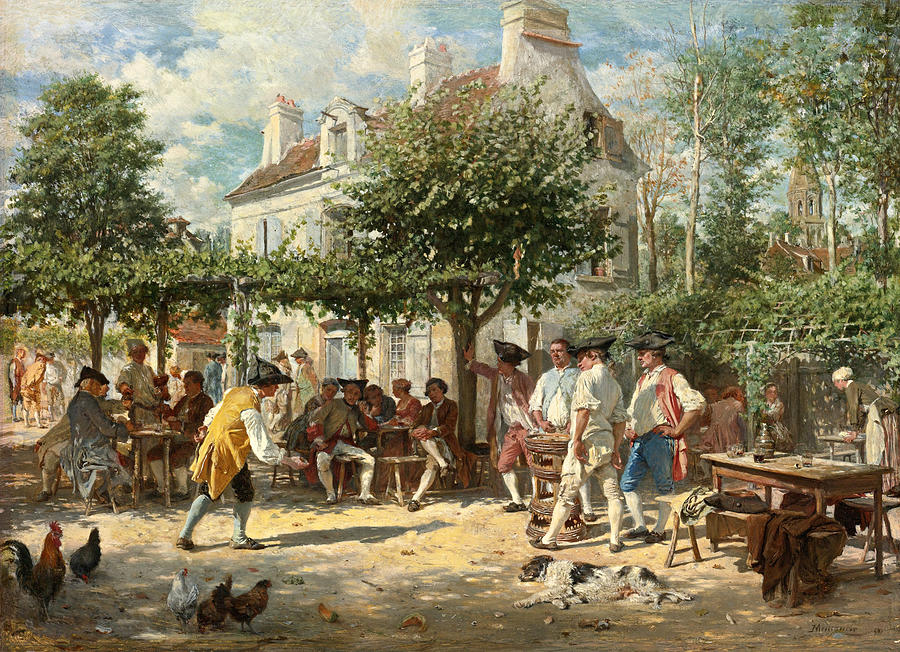This detailed painting, set in an outdoor space reminiscent of Colonial or Revolutionary times, showcases a vibrant scene near a large house with a reddish roof and chimneys. Surrounding the wooden tables are men dressed in traditional attire, including knickers, long vests, and white shirts with tricorn hats. One man stands out in blue pants with a white shirt and red vest, while another wears a gold vest. In the foreground, a black and white cocker spaniel lies in a sunbeam, and several roosters and chickens, including a red and green rooster, mill about. An apple tree is positioned centrally in the background, with tall trees framing the scene, all set under a blue sky scattered with clouds.